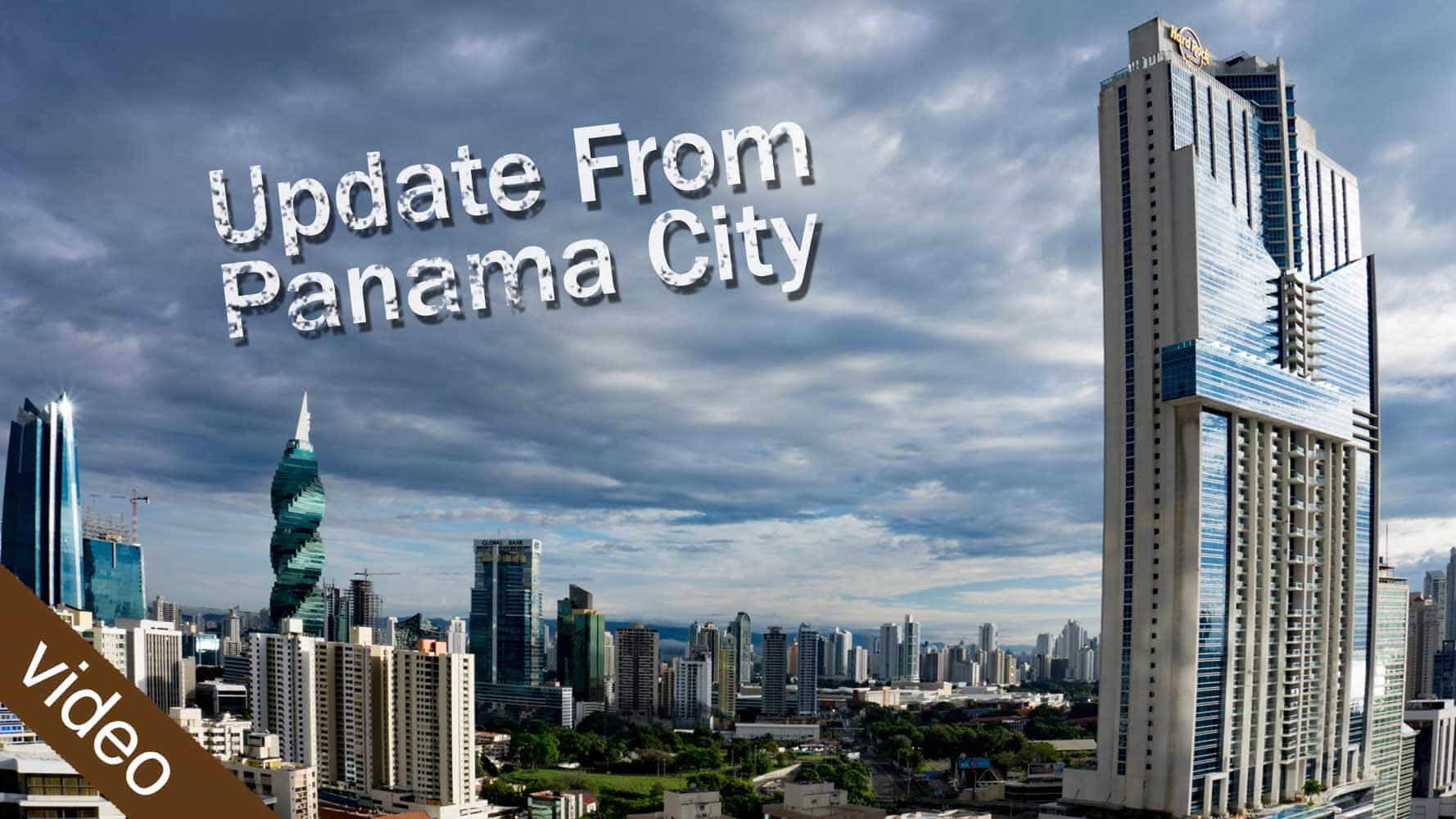A screenshot from a computer captures a panoramic cityscape under a bluish-gray sky. The top three-quarters of the image is dominated by the expansive sky, with clouds concentrated in the upper half. In the image's center, bold capital letters declare: "UPDATE FROM PANAMA CITY." In the bottom left corner, a brown sideways banner indicates this is a video.

The foreground prominently features an array of skyscrapers. On the far right, a towering silver building stretches from the bottom to the top of the frame, viewed almost side-on. At its peak, a yellow "Hard Rock" sign is visible. Towards the middle of the skyline, most buildings reside just below the horizon. One notable structure, with a twisted, spiraled architecture and a pointed tip, stands out. To its left, another large silver building catches sunlight on its upper levels.

At the bottom center, a patch of greenery with trees is visible, adding a touch of nature to the urban vista.